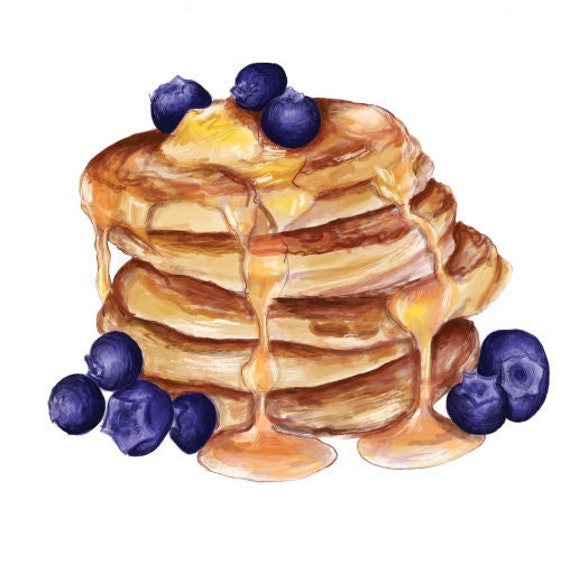This is a detailed illustration of a delicious stack of pancakes, consisting of six slightly off-center, perfectly baked, thick, and gooey pancakes. Each pancake displays a rich, brown sheen, indicative of perfect cooking. Atop the stack sits a generous glob of golden butter, which has started melting and cascading down the sides. Adding a colorful contrast are three dark purple blueberries positioned in the center of the top pancake. Maple syrup has been lavishly poured over the stack, soaking the top layer and creating a beautiful, sticky cascade down the sides, pooling at the bottom in a golden glob. Surrounding the stack at the base, on the left side, are four more blueberries, while the right side features two additional blueberries. This eye-watering stack looks irresistibly yummy, with the syrup, butter, and fruit combining visually to create a mouth-watering breakfast treat.